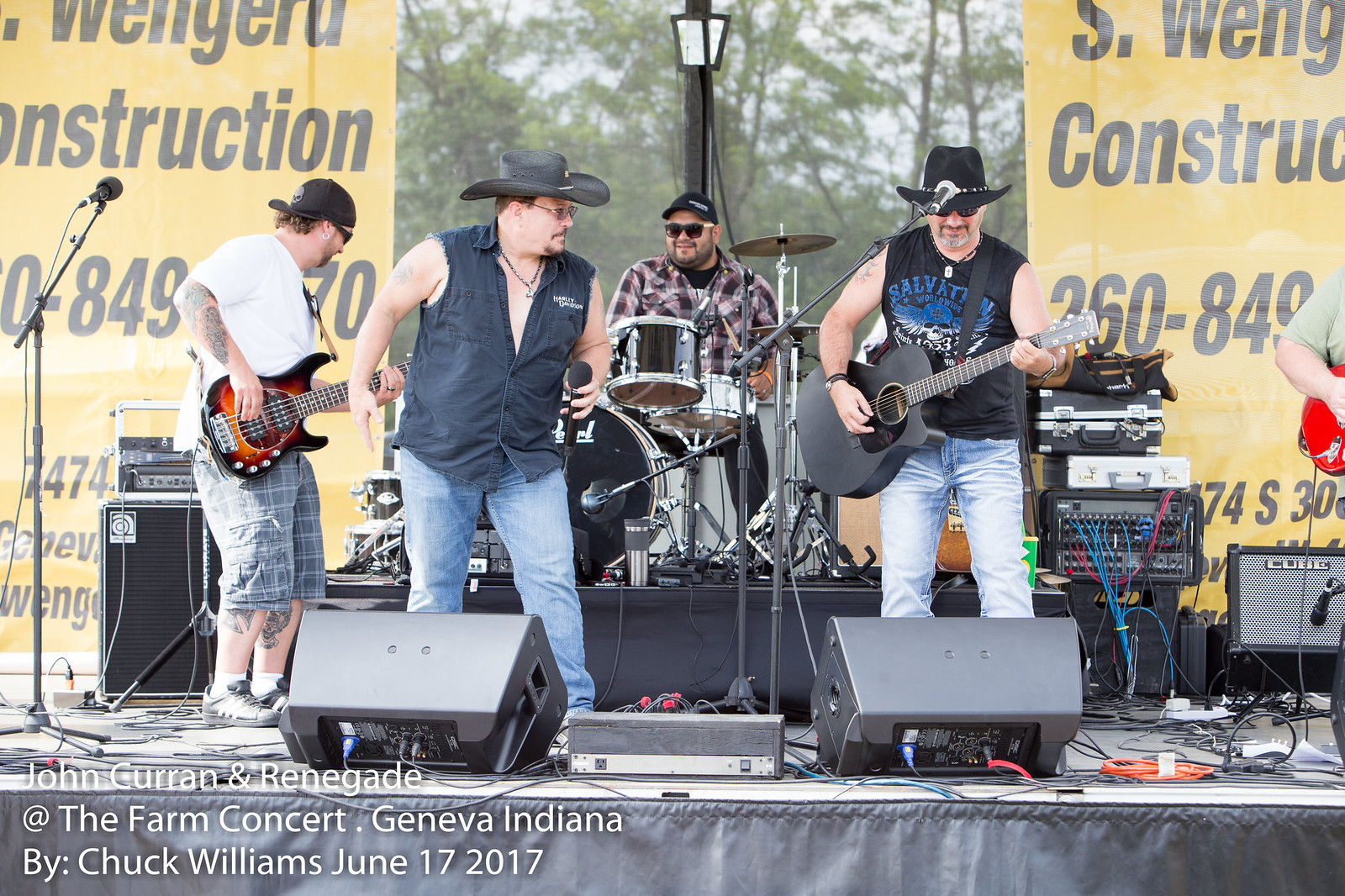This photograph captures an outdoor concert stage featuring the band "John Gruen and Renegade" at the Farm Concert in Geneva, Indiana, taken by Chuck Williams on June 17, 2017. On the stage, there are four primary musicians and a partial view of a fifth person, identified by an elbow and a red electric guitar on the far right. At the front of the stage, two men in sleeveless black shirts and blue jeans – both wearing dark-colored cowboy hats – take the lead. The man on the right wields a black guitar, while the one on the left holds a microphone. Immediately behind them, another man in a white shirt, black backward baseball cap, and plaid shorts adorned with numerous tattoos plays an electric guitar, facing slightly away from the audience. At the very back, the drummer, clad in sunglasses, a black hat, and a plaid shirt, sits behind his drum set, flanked by electronic equipment. Two yellow signs with black writing, promoting "S. Wengerd Construction," are visible on either side of the stage with a backdrop of trees. The caption at the bottom left-hand corner of the image reads, "John Gruen and Renegade at the Farm Concert, Geneva, Indiana by Chuck Williams, June 17, 2017."